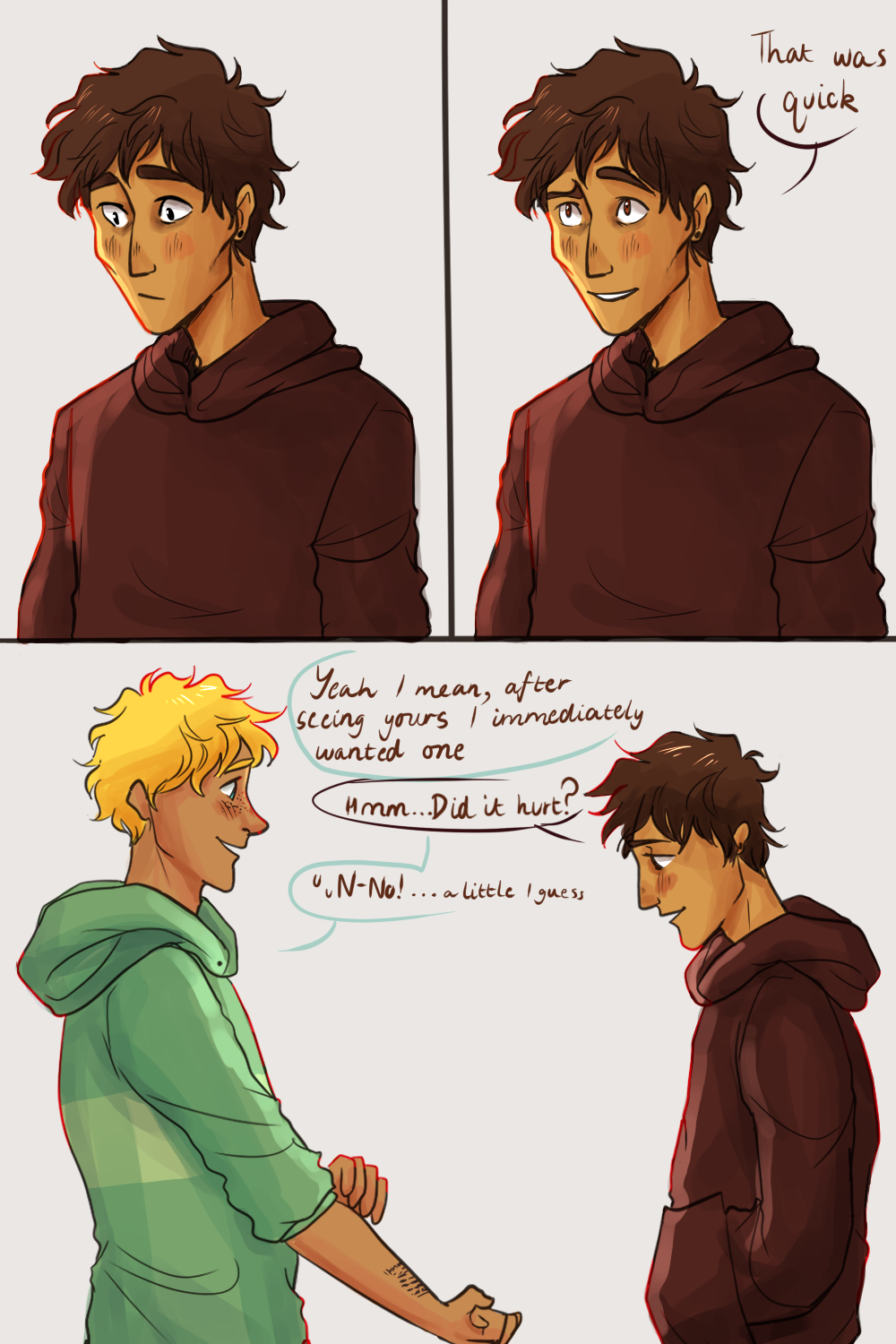The image features two distinct sections of sketched cartoon characters. At the top, there are two illustrations of a character divided by a black vertical line in the center. On the right side of this section, a character with short brown hair, styled longer than a buzz cut, is wearing a brown hoodie sweatshirt and saying "That was quick." The background is light gray.

In the bottom section, the setting continues with a light gray background, showcasing a conversation between two characters from a side view. The character on the right, still wearing the brown hoodie, responds, "Yeah, I mean, after seeing yours I immediately wanted one. Hmm, did it hurt?" On the left, the other character, who has blonde hair and is wearing a green hoodie with rolled-up sleeves, answers, "No," while pointing to a small tattoo on his wrist, which appears to be the topic of their discussion.